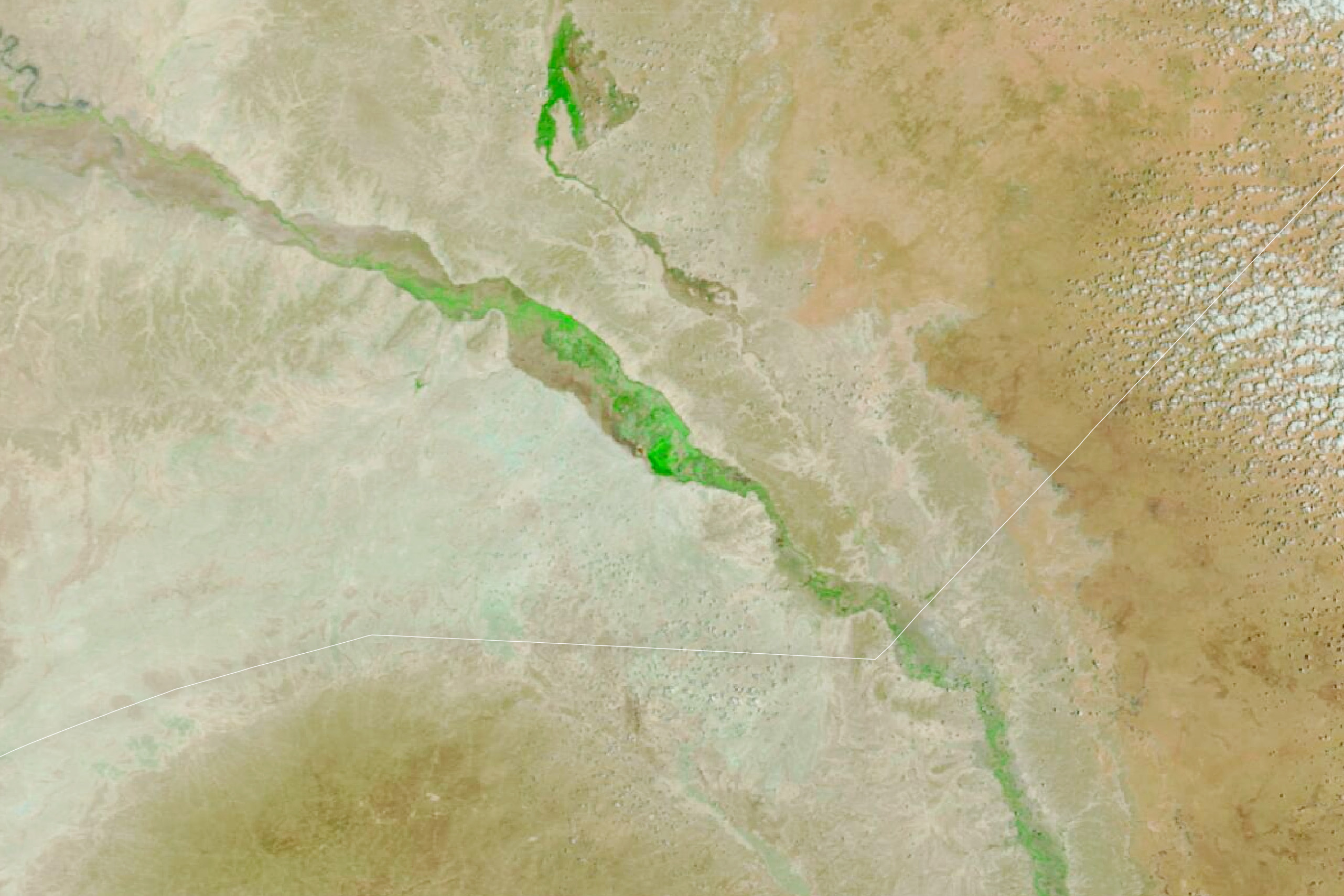This image is a fascinating close-up that appears to be a detailed depiction of a terrain or a painting. The left side of the image begins with shades of white and gray, gradually transitioning to darker shades of orangey or greenish-brown as you move towards the bottom. Towards the far right, light tan and blotchy light green areas emerge, with highlights reflecting light, possibly resembling the textured pores of leather or skin. 

A distinct feature is a tan line starting from the top left corner, evolving into a vivid green color as it stretches diagonally across the image towards the bottom right. This line might represent a geographical element such as a ridge or river. The top right corner shows pitting or a powdered substance, adding to the textured look. 

Hints of green are scattered throughout, particularly towards the top center and upper side, enhancing the earthy palette dominated by gray and sandy brown shades. The overall pattern of colors ranges from light brown to dark gray, interspersed with green, suggesting a natural landscape, possibly a desert or mountain region, captured in an abstract or aerial view.